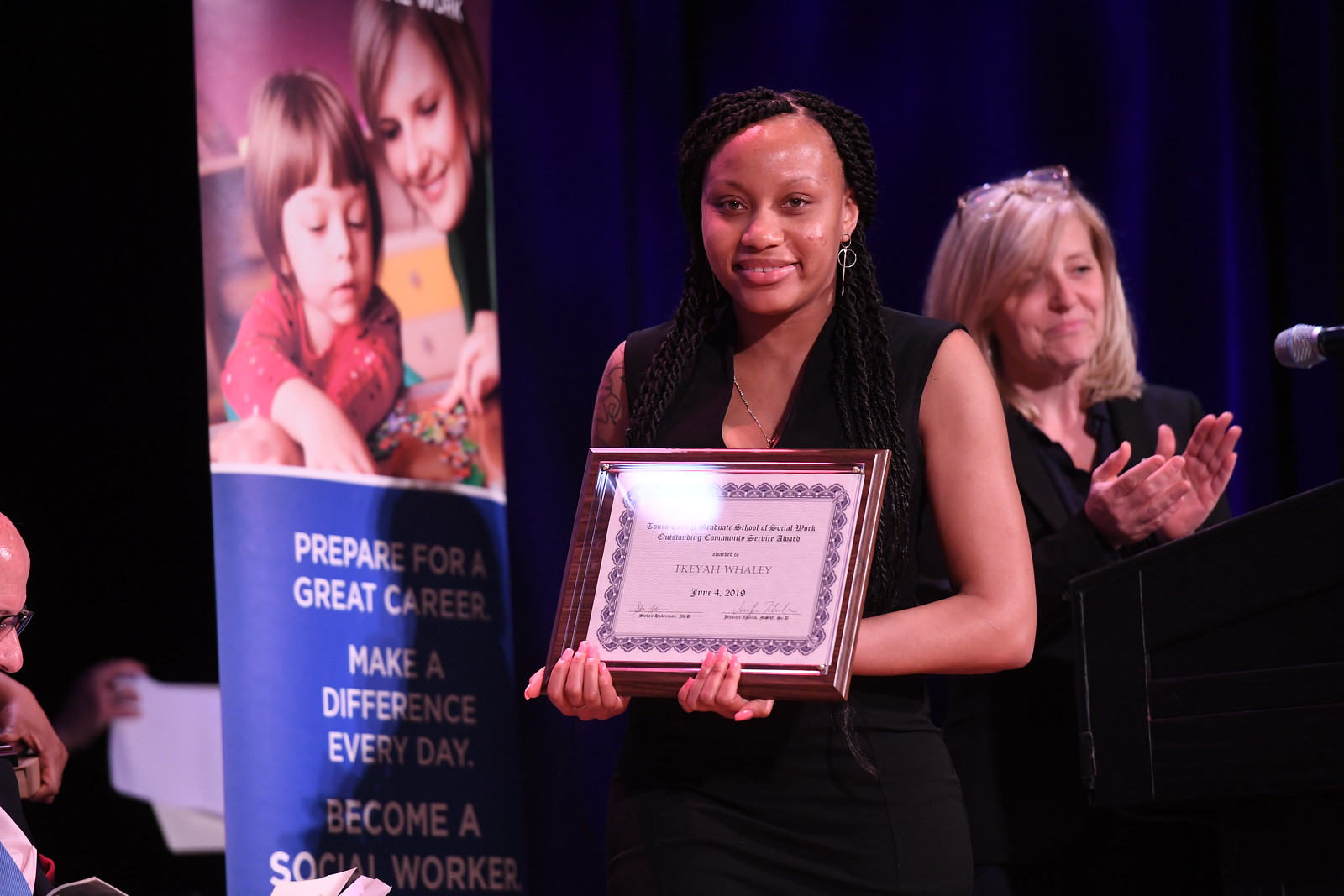In the image, we see an African-American woman in her 20s wearing a sleeveless black dress, smiling as she holds an Outstanding Community Service Award plaque in front of her torso with both hands using an underneath grip. Her hair is styled in dreadlocks, and she sports a dangling earring in her left ear along with a tattoo on her right arm. The plaque, dated June 4, 2019, identifies her as Takia Whaley. Standing to her right is a dirty blonde-haired white woman, who has glasses perched on top of her head and is clapping her hands while standing behind a podium with a microphone, presumably announcing the award. The background features a dark blue curtain and a promotional banner depicting a white woman with a child. The banner's lower half is blue with white text that reads, "Prepare for a great career. Make a difference every day. Become a social worker." This setting suggests a ceremony recognizing women for achievements in social work.